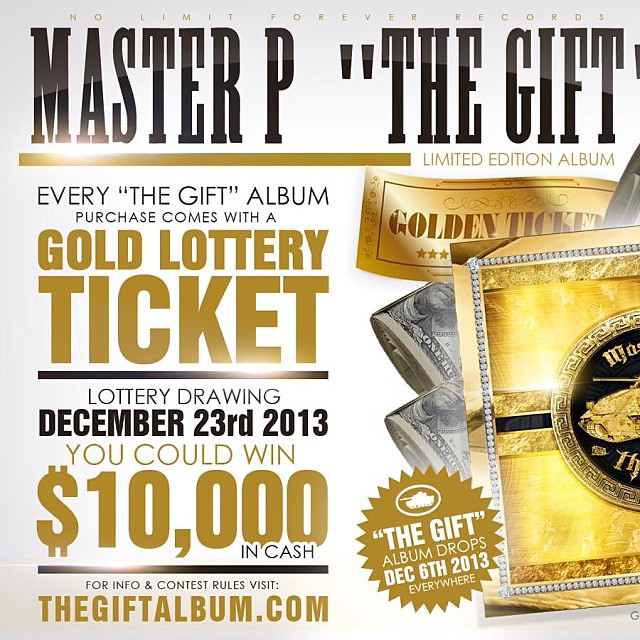The advertisement for Master P's "The Gift" album features a prominent white square background with bold, black text at the top reading "Master P." Directly beneath this, in the same black font but enclosed in quotation marks, is the album title "The Gift." Above this text, in small gold letters, the phrase "No Limit Forever Records" is displayed. Below the album title, a horizontal gold bar separates the sections, followed by the gold text "Limited Edition Album."

Further down, a detailed promotional message in black font states that every purchase of "The Gift" album includes a gold lottery ticket, with "gold lottery ticket" accentuated in large, gold letters. Underneath, a black line divides the message, which continues with details about a lottery drawing on December 23, 2013. Following this, in gold text, it highlights the potential to win $10,000 in cash. Additional information in black font directs viewers to visit TheGiftAlbum.com for more details and contest rules.

On the right side of the image, a visually appealing graphic showcases a golden ticket, accompanied by rolls of $100 bills partially concealed by a lavish gold emblem adorned with diamonds. An overlaying gold seal with white text declares, "The Gift Album Drops December 6, 2013, Everywhere," adding a final call to action. The visual elements reinforce the luxurious and exclusive nature of the album release.